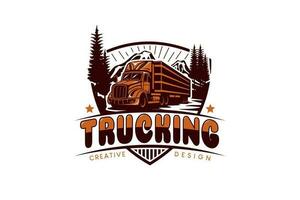The image is a compact logo set against a solid white background without any border. Central to the design is a brown semi-truck, which dominates the scene with its elongated depiction. The truck is set above the word "TRUCKING," which is written in bold, bubble letters. These letters are colored in a gradient, transitioning from medium brown at the top to black at the bottom. Adding depth to the image, there are two subtly curved black lines flanking the word "TRUCKING."

Surrounding the truck are nature elements that frame the design: on the left side, two overlapping pine trees outlined in black, and on the right side, a couple more pine trees positioned behind the truck. In the background, a delicate outline of mountains stretches across, providing a scenic backdrop. Below the bottom curved line, there's a triangular shape appended, adorned with vertical lines.

At the base of the logo, the words "CREATIVE DESIGN" are displayed, written in gold-colored, all-capital, sans-serif font. The overall composition is detailed and clear, showcasing the truck and text prominently against the bright, uncluttered white setting.